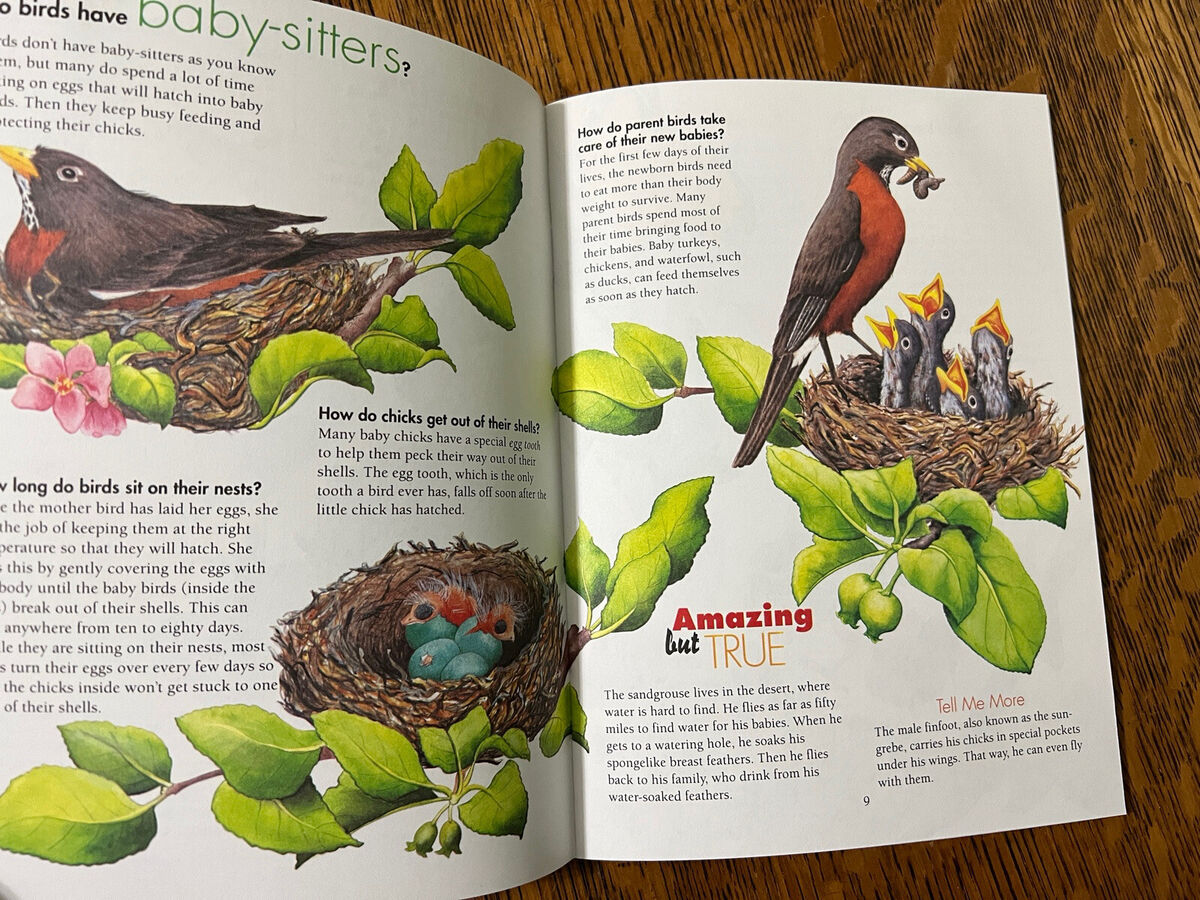The photograph showcases an open book placed on a rich, dark brown, wooden surface adorned with prominent, darker diagonal grain lines. The book, likely designed for children, focuses on avian life and features white pages filled with black text and vivid illustrations. The left page, partially cropped, is titled "Do birds have babysitters?" and is accompanied by an image of a bird in a nest surrounded by trees. This page explains various aspects of bird life, including how birds care for their eggs and chicks, with paragraphs discussing topics like egg incubation and the hatching process. The right page, numbered 9, is fully visible and features a colorful illustration of a mama bird, probably a robin, feeding its baby birds, with detailed scenes including another nest with eggs and newly hatched chicks. Three distinct paragraphs break up the text, which appears on the upper left, lower left, and lower right, detailing the nurturing behaviors of birds. The combination of informative text and engaging images serves to educate young readers about the fascinating lives of birds.